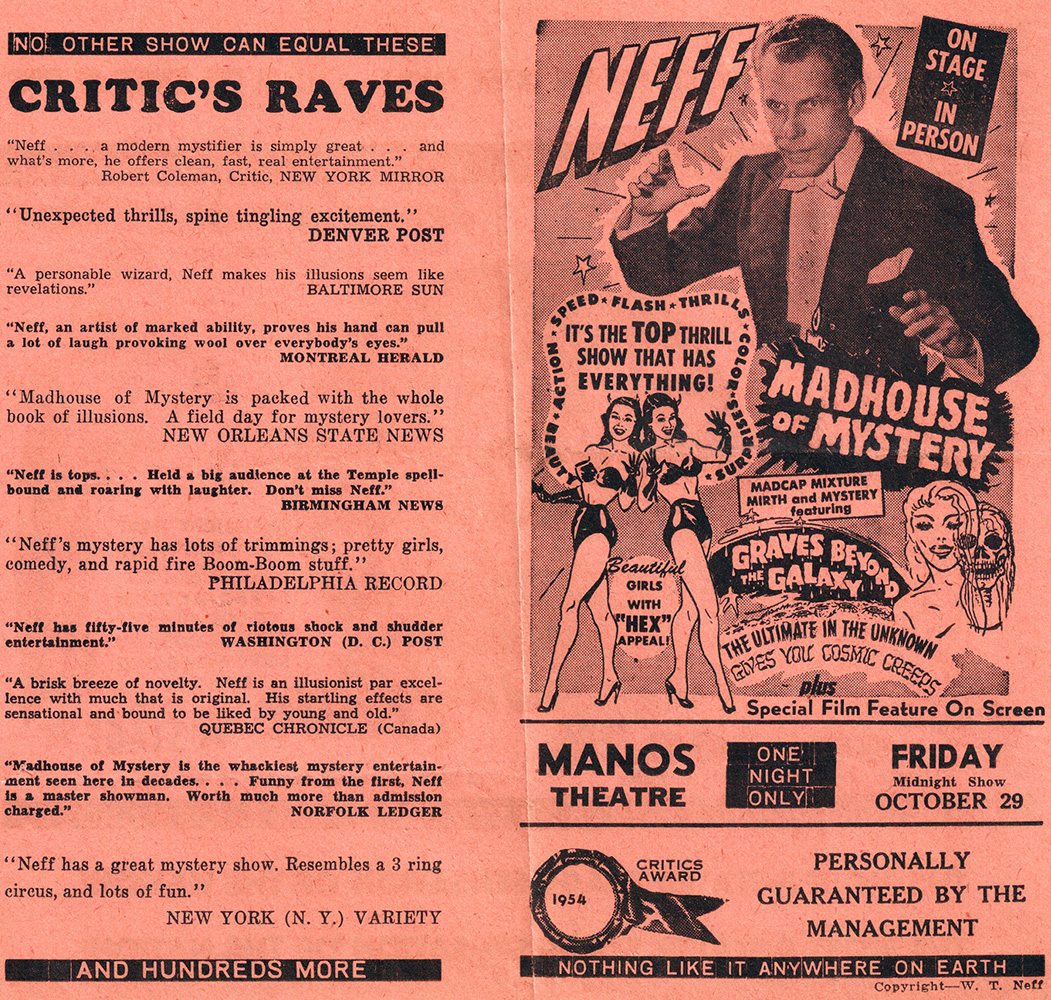This detailed image showcases an old theater show program brochure from the Mantos Theater featuring the "Madhouse of Mystery," headlined by Neff, a classic magician. The pamphlet, which appears to be in a color spectrum between dark pink and lightish red, potentially peach, is printed on heavy stock paper with a notable crease indicating it was once folded. 

On the left side, the tagline "No other show can equal these critics' raves" catches the eye, displayed in prominent black text. Below this, there's an array of enthusiastic reviews from various notable sources. One highlighted review from the New York Mirror states, "Neff, a modern mystery, is simply great, and what’s more, he offers clean, fast, real entertainment," attributed to critic Robert Coleman. Another review from the Denver Post heralds "unexpected thrills, spine-tingling excitement." At the bottom of this section, surrounded by a black box, is the claim, "and hundreds more," printed in a font that blends into the background color.

On the right side, we see the main attraction: an image of Neff, dressed in a black jacket and peach-colored bow tie, posing dramatically with his hands raised, giving a classical magician's flair. Above him, the brochure proudly displays "Neff," and to his right, it announces "on stage in person." Below Neff, the bold title "Madhouse of Mystery" is presented. Adjacent to Neff's image are two women dressed in black bras and short shorts, with a caption reading, "It’s the top thrill show that has everything—beautiful girls with hex appeal." Further down, there’s an eerie illustration of a woman with a skull beside her, under the text "graves beyond the gallery—the ultimate in the unknown gives you cosmic creeps."

The bottom section provides logistical details, noting a special midnight show at the Mantos Theater on Friday, October 29th, 1954, with a confident endorsement: “Personally guaranteed by the management. Nothing like it anywhere on earth.” Additional markers like copyright WTNF are also visible, emphasizing the unique and historical aspect of the show.